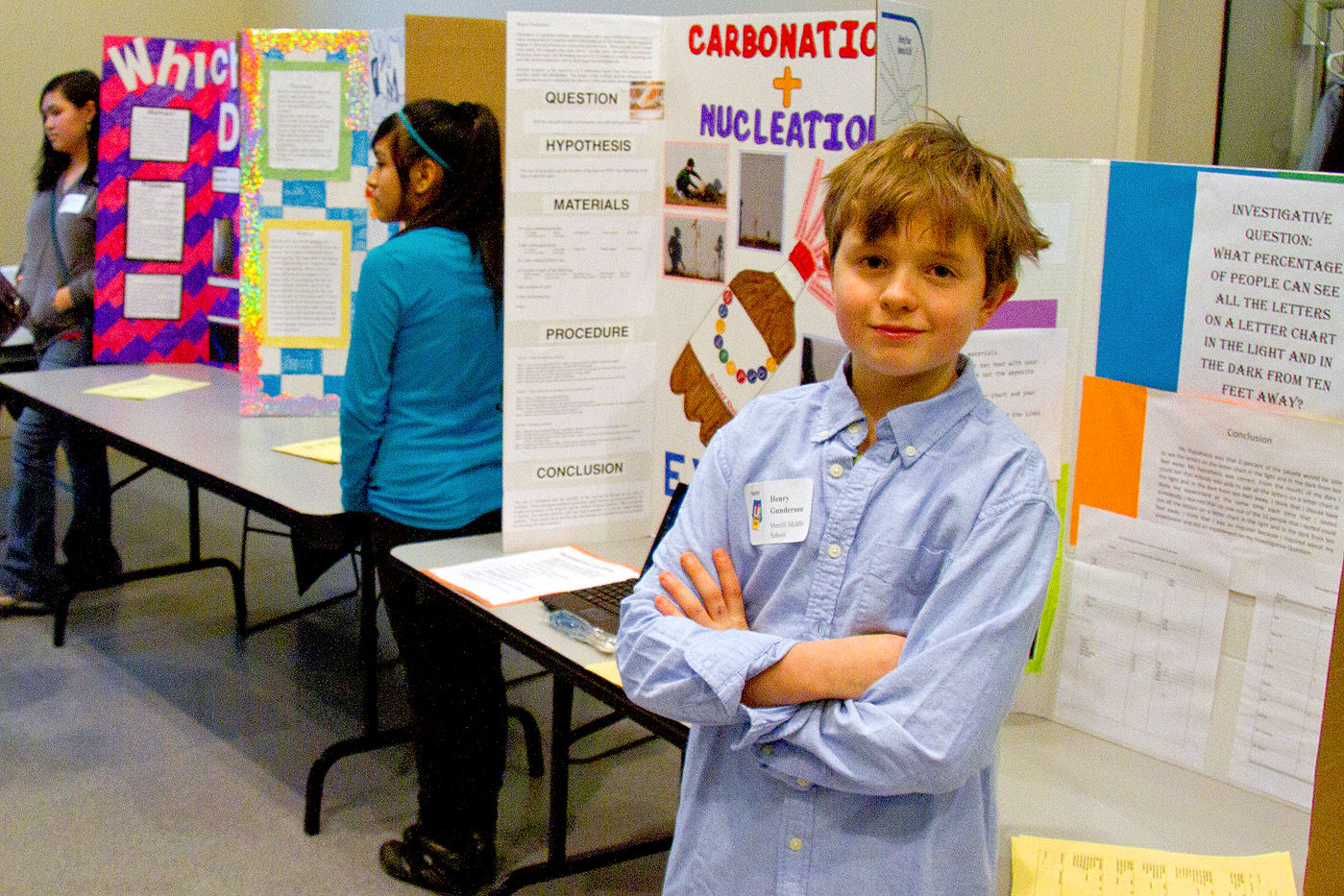In this vibrant photograph from a junior high school science competition, a cheerful young boy stands proudly in the foreground, arms crossed and smiling directly at the camera. He sports a blue shirt, a neat white badge, and tousled brown hair. His investigative project poster behind him explores the intriguing question, "What percentage of people can see all the letters on a letter chart?" Next to him, a girl dressed in black pants and a matching blue shirt looks away, absorbed in her own project. The background bustles with white tables lined with diverse science projects, their posters rich with colorful text and imagery detailing questions, hypotheses, materials, procedures, and conclusions. Another participant in a light blue headband and shirt is visible in the background, alongside a third contestant in a gray shirt and jeans. The school setting is filled with hues of red, purple, yellow, peach, white, black, and gray, all underpinned by the excitement and curiosity of budding young scientists.